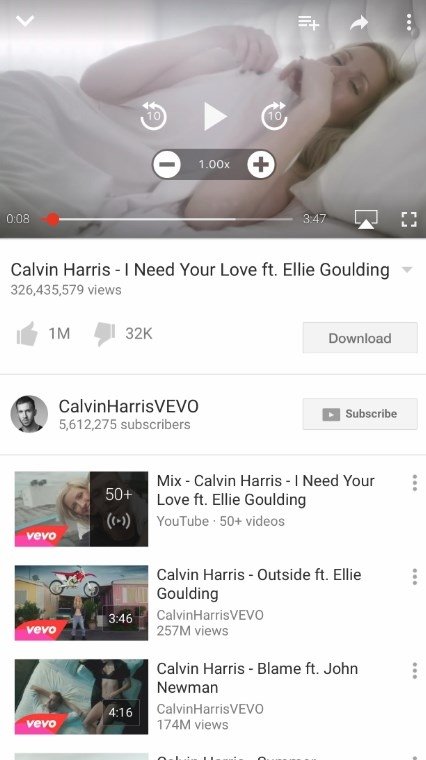This image depicts a screenshot of a YouTube video featuring a woman lying in bed, seemingly in distress or possibly crying. The video player interface is visible, showing a progress bar currently at 8 seconds into the video, indicated by a red dot on a white line. The total duration of the video is 3 minutes and 47 seconds. The video is a music clip titled "Calvin Harris - I Need Your Love ft. Ellie Goulding" and has garnered millions of views. It has received approximately 1 million upvotes and 32,000 downvotes. Below the video, there are options to download the video, subscribe to Calvin Harris's channel, and explore additional content. Three more related video thumbnails are displayed, including "Calvin Harris - Outside ft. Ellie Goulding" and "Calvin Harris - Blame ft. John Newman."